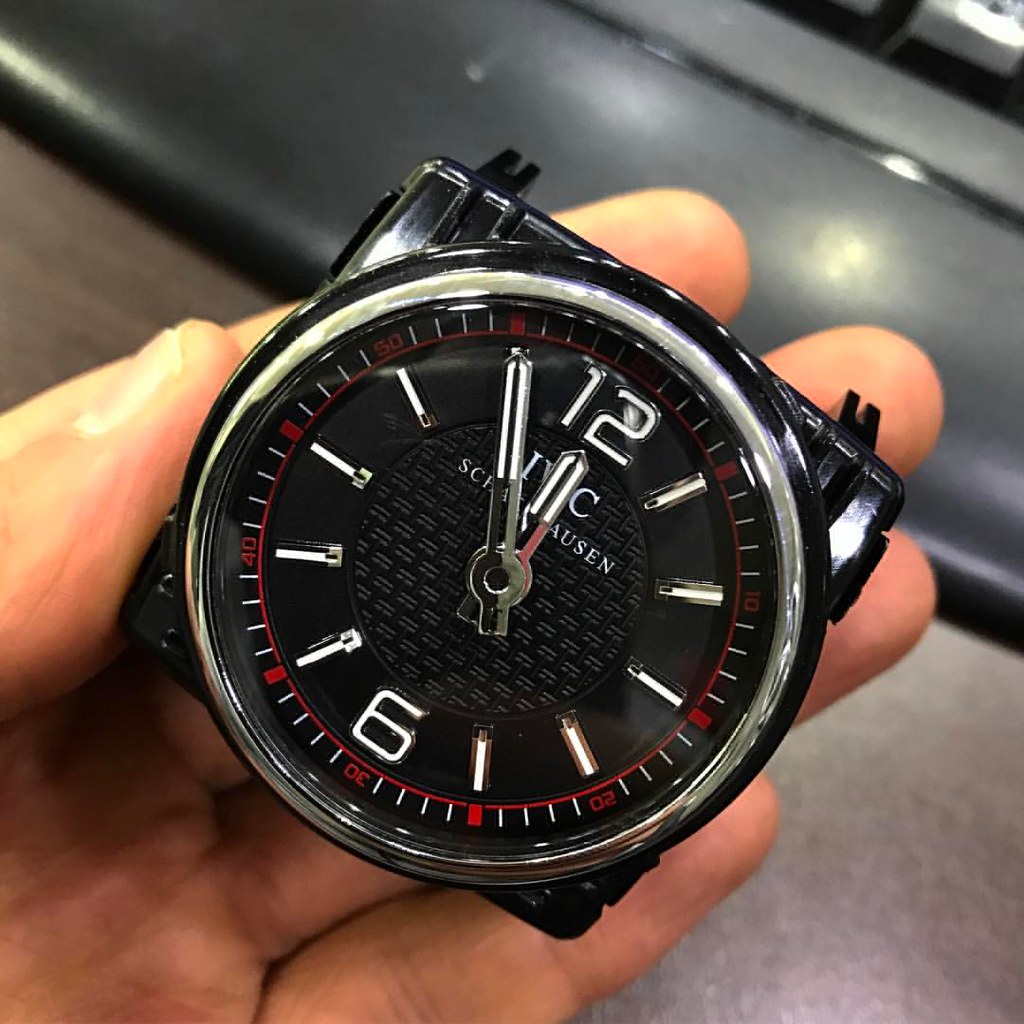Caption:  
In this detailed close-up shot, a hand firmly grips a stylish black watch with a thick, angular face. The thumb is positioned on the left side of the watch, while three fingers support it from behind, with the pinky stabilizing the corner edge. The watch's design features prominent white numerals at the 12 and 6 o'clock positions, and silver hands with white strips on either side, allowing them to glow in the dark. Additional white strips mark each hour. Red cubes encircle the outer rim, along with a full set of numerals. The watch is held above a brown table, and a leather object is partially visible in the background on the right. The entire watch face is angled towards the top right corner, adding a dynamic element to the composition.